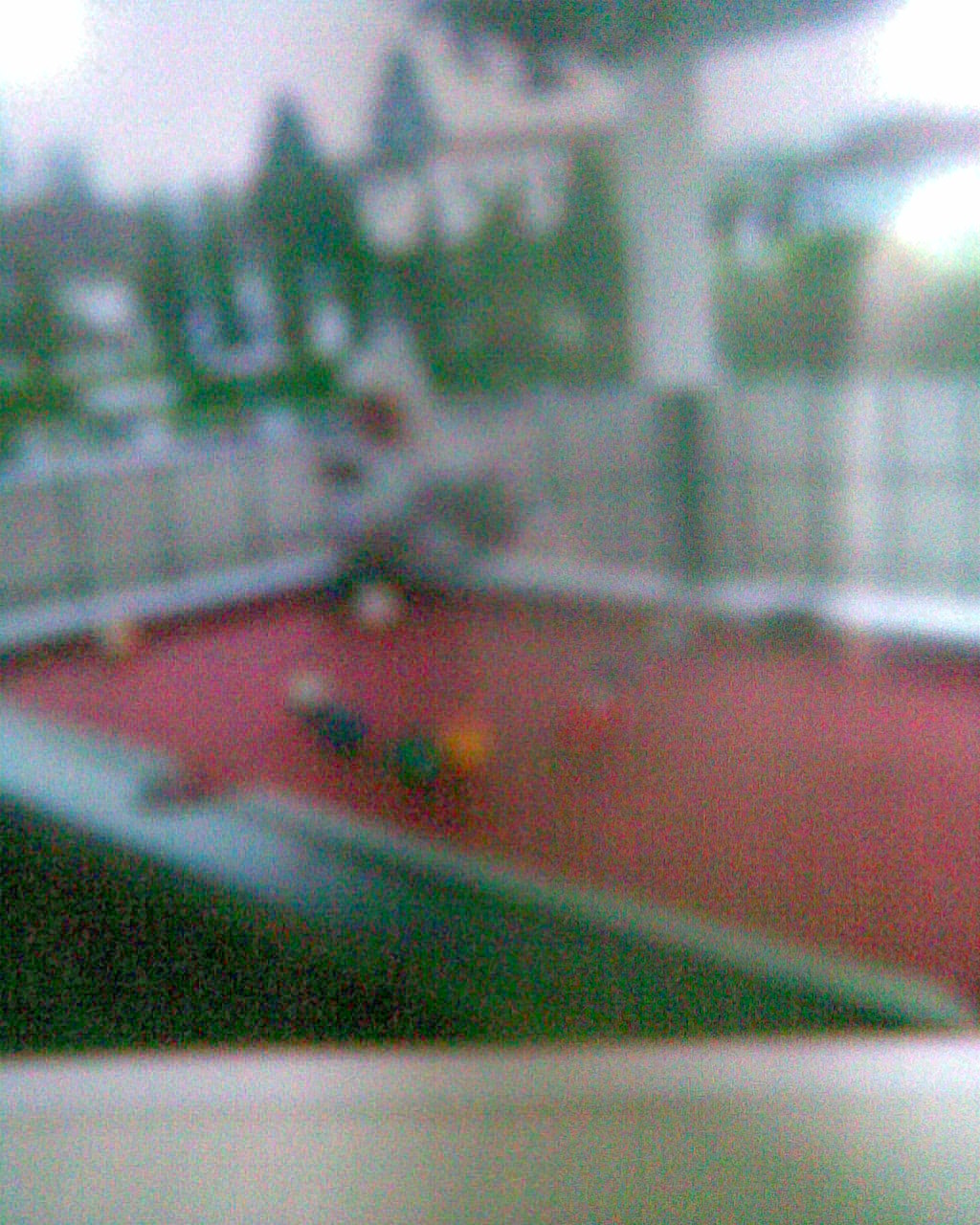A blurry photograph capturing a daytime scene on a deck or porch in a residential neighborhood. The focal point is a pool table with a green playing surface and a red tabletop. On the table, there are at least six pool balls visible, although out of focus. A person is present in the image, positioned behind the cue ball and appearing to lean their elbows on the table. The background reveals trees and neighboring homes, adding to the suburban ambiance.